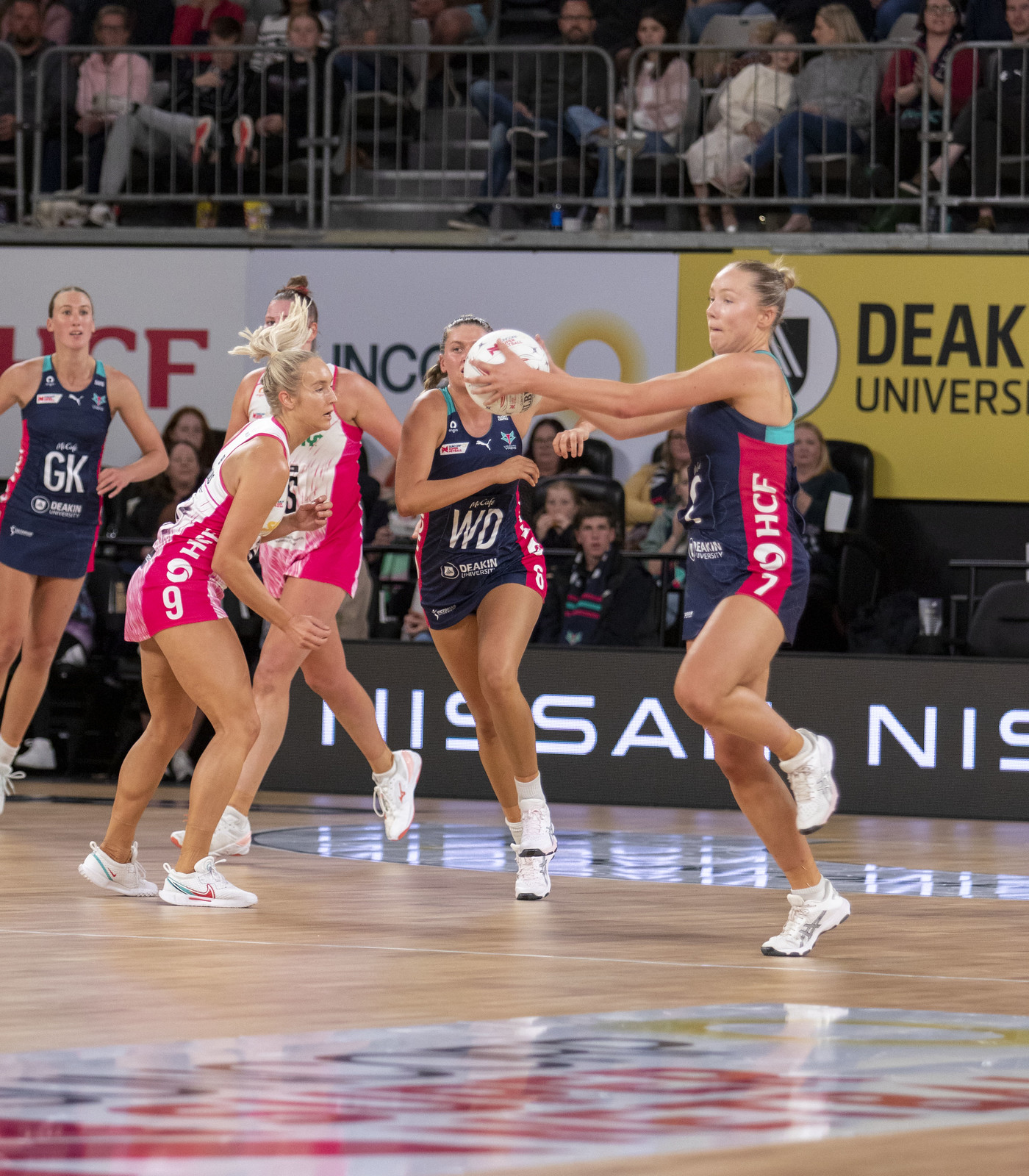The image captures an intense handball game taking place on an indoor hardwood court, marked with sporting lines and sponsor logos, including a noticeable "Nissan" banner. The game features five tall women, divided into two teams distinguished by their uniforms. Three players wear navy blue tank tops with red and green stripes, paired with blue shorts with red stripes. The other two athletes sport white uniforms accented with hot pink stripes. All players are equipped with white sports shoes, likely from Nike. On the far right, one player is holding the ball, while the other four are poised and moving towards it, suggesting dynamic gameplay. Notably, one player's uniform is marked with "GK," indicating her role as the goalie. In the background, an enthusiastic crowd is visible, seated in a stadium setting with gray steps leading up to the seating area, adding to the excitement of this indoor sporting event.